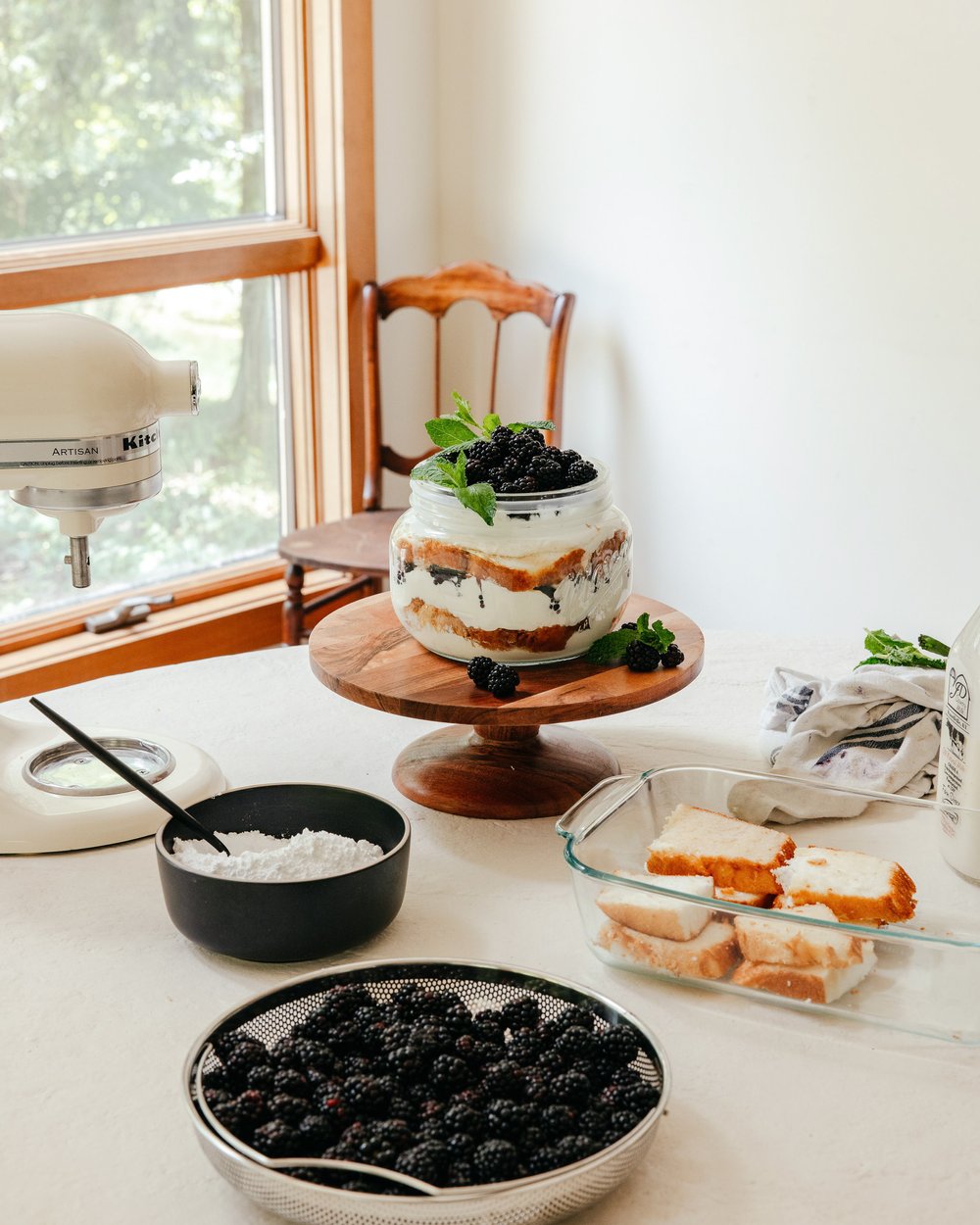The indoor photograph captures a white round table adorned with various kitchen items organized for baking or preparation. Centered on the table is a one-tiered wooden stand displaying a large decorative jar filled with spongy bread or a parfait-like mixture featuring blackberries on top and leaves as garnish. Just in front of the stand, towards the bottom of the image, a small wired strainer overflows with fresh blackberries, positioned slightly to the left. Beside the strainer sits a black bowl filled with what appears to be flour and a black spoon inserted into it. To the right of this arrangement, an oval glass baking dish contains around eight slices of what looks like pound cake. The background reveals a cozy kitchen with a wooden chair and a window casting natural light onto the scene. Additionally, on the far right of the table, a used rag and a jar of milk are visible, contributing to the authentic kitchen ambiance.